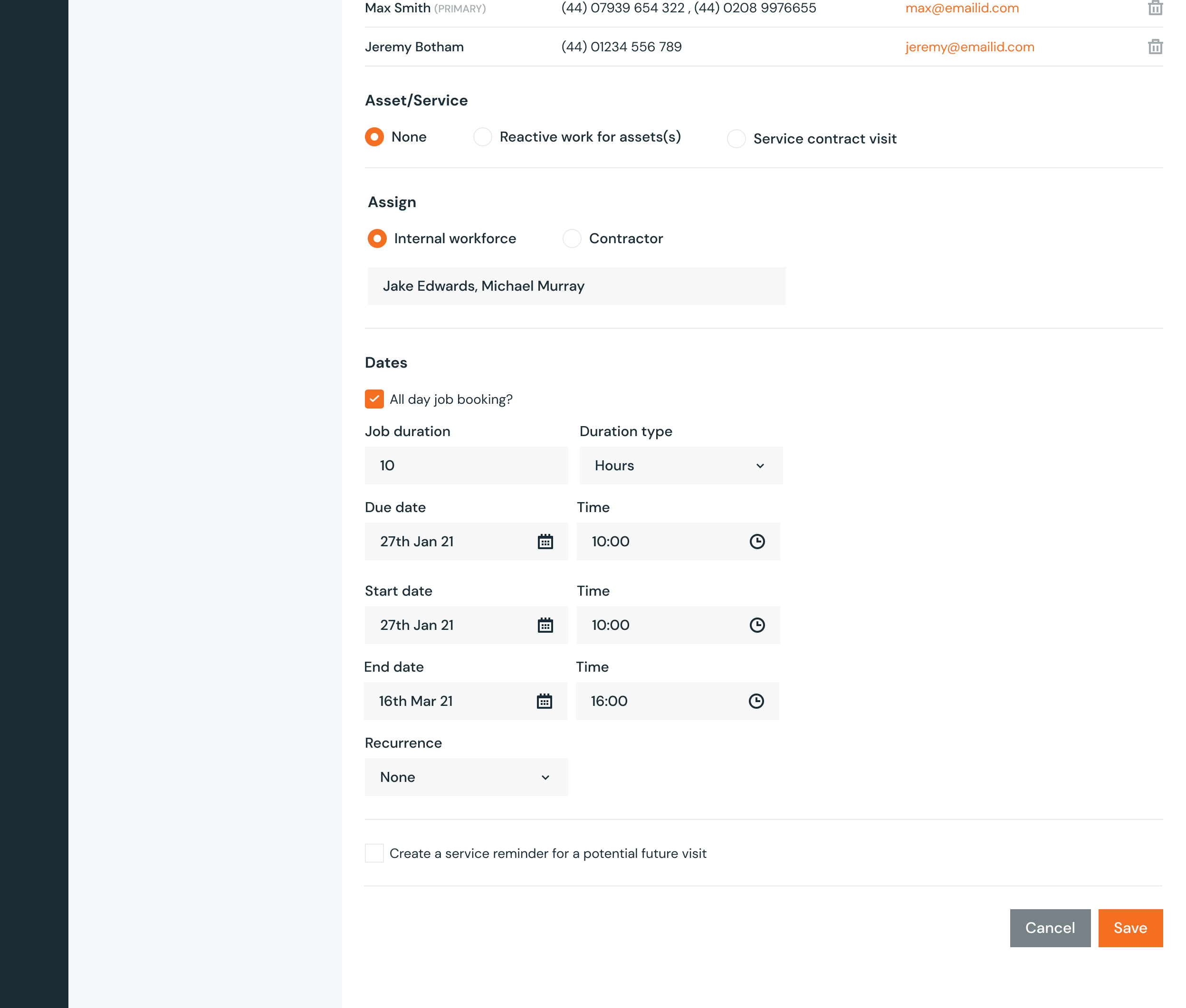This image is a screenshot of an application interface with a predominantly white background and black text. There are additional elements in a rust-colored or orangey-rust hue. On the far left edge, a bold black stripe contains various data entries. 

**Max Smith** is the first entry, with the label "Primary" grayed out next to his name. His telephone number and email address are displayed, with the email address highlighted in orange. A delete icon in the form of a trash symbol is also present for this entry.

**Jeremy Botham** follows as the second entry, displaying his telephone number and email address in the same orange hue, accompanied by the same delete icon.

Below these two entries, the label **"Asset/Service"** is bolded. An orange circle with the word **"None"** beside it is noted under a sub-section labeled **"Reactive Work for Assets, Service, Contract Visit."**

Further right, there are two categories: **"Assign"** and **"Dates."** The **"Assign"** category is followed by the **"Dates"** category, detailing information related to all-day job bookings and job duration.

The layout and displayed data suggest that the app is designed to track various tasks and assignments for the indicated individuals, providing a structured overview of their jobs and schedules.